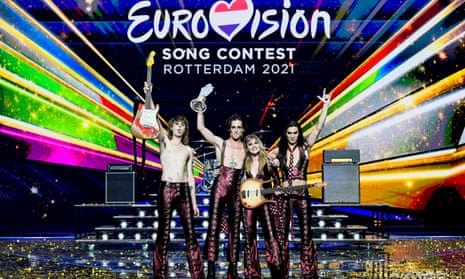The image captures a jubilant scene at the close of a Eurovision event, specifically the Eurovision Song Contest 2021 held in Rotterdam. The "Eurovision" title is prominently displayed at the top, with a creative mix of uppercase and lowercase letters—the first half in all caps transitioning to mostly lowercase. The letter 'V' is charmingly replaced with a red heart symbol, signifying love and unity. The colorful logo features a tricolor design: the top third in vibrant red, the middle third in white, and the bottom third in a purplish-blue hue. Below, the text "SONG CONTEST" is written in sleek, all-capital letters.

The spotlight is on a victorious band, consisting of four members who appear in matching outfits. The second member from the left proudly holds up a trophy indicating their triumph. The band member on the far left hoists a guitar in celebration. The person on the far right displays a classic rock-and-roll hand gesture, adding to the festive mood. The only woman in the group, positioned third from the left, casually rests a guitar by her side. 

Behind them, a multi-tiered platform with steps houses drum sets in the center and sound equipment on the sides. The stage backdrop features an array of dynamic light bars emanating from the top left and right corners, converging towards the center, enhancing the electrifying ambiance of the event.